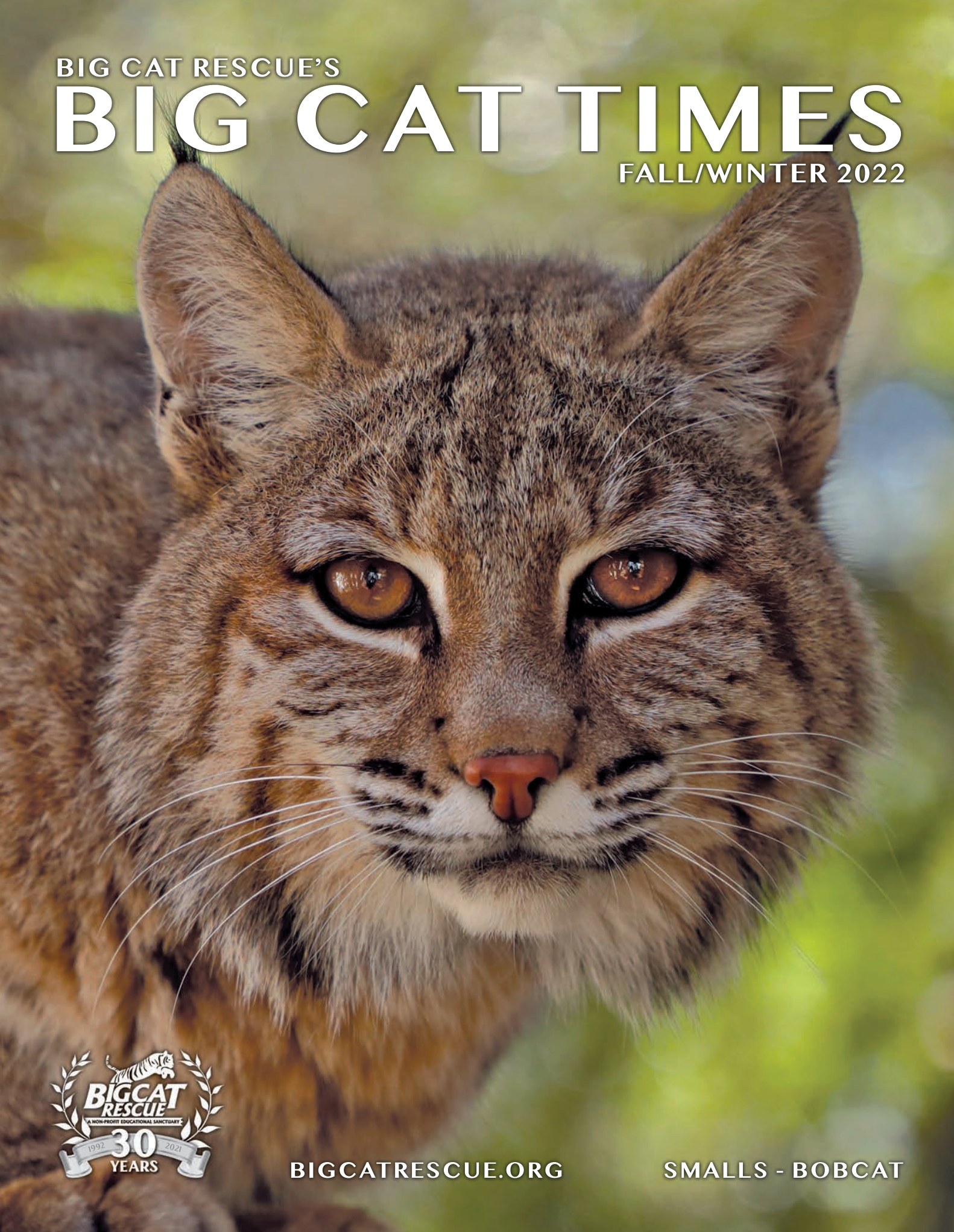The cover of the Fall-Winter 2022 issue of "Big Cat Times," titled "Big Cat Rescues," features a close-up photograph of a bobcat named Smalls. The bobcat, with its orangey-brown fur and striking orangey-brown eyes, looks straight into the camera, capturing attention with its intense gaze. Its nose, a distinct reddish hue, contrasts with the primarily brown and white fur. The background features a blurred mix of green and blue, emphasizing the bobcat's face. In the bottom left corner, an emblem celebrating 30 years of Big Cat Rescue shows a jumping tiger surrounded by a banner and decorative leaves. Beneath the emblem, the website "BigCatRescue.org" is printed in white, along with "Smalls-Bobcat."